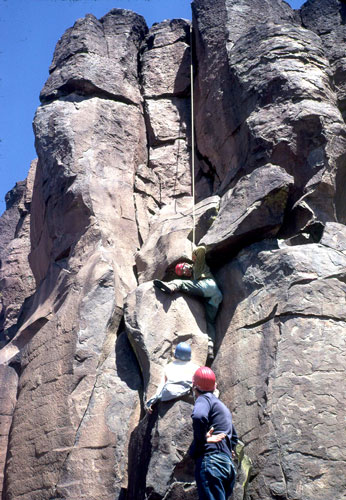In this detailed and vivid photograph of an exhilarating mountain climbing scene set against a clear blue sky, a rugged rock face occupies most of the frame. A long rope descends from the top of the cliff, aiding the climbers. On the ground, a man with a red helmet, navy blue t-shirt, and blue jeans stands with his left arm braced on his hip, leaning against the boulders. Nearby, another man wearing a blue helmet and light blue shirt gazes upward. Higher up the rock face, a climber with a red helmet and one leg propped on a boulder looks down at the two men below. His body is contorted as he navigates a crevice, lifting one leg while gripping the rope. This dynamic scene showcases the intense focus and coordination of the climbers as they conquer the challenging terrain.